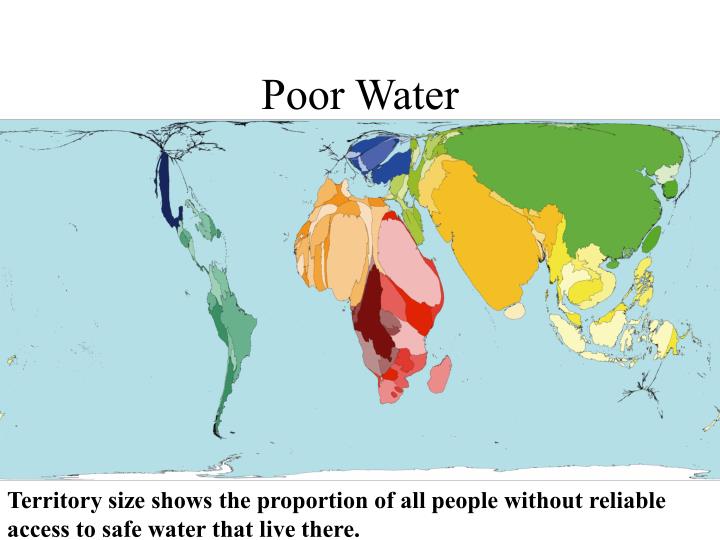The image is a vibrant, flat, clipart-style world map, designed as an infographic to depict global water insecurity. The continents are distorted in size to represent the proportion of people without reliable access to safe water within each territory. At the top of the map, in black and white text, "poor water" is prominently displayed, with "poor" spelled "P-O-O-R." 

Each continent is color-coded: the United States in dark blue, South America in sage green, Africa shaded in red and orange, the China area in forest green, Europe in baby blue, and the Middle East in yellow. The color palette ranges from dark red to aqua blue. 

Despite some blurriness and skewed shapes making specific countries difficult to identify, the image effectively communicates its message. The bottom of the illustration includes a caption explaining, "Territory size shows the proportion of all people without reliable access to safe water that live there."